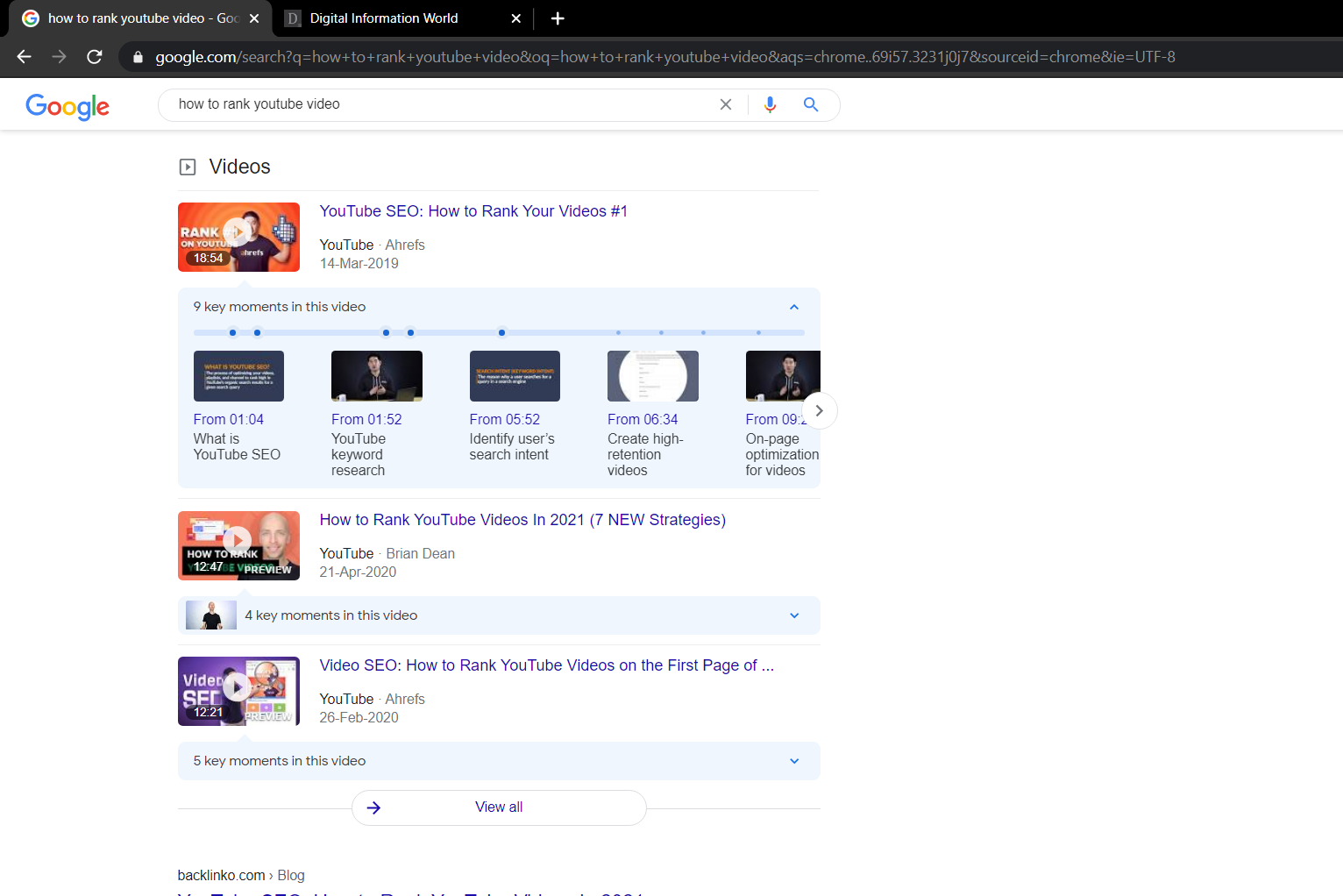A screenshot of Google search results focused on how to rank YouTube videos. The page displays multiple entries on YouTube SEO, including topics like keyword search, user search intent, creating high retention videos, and on-page optimization. Specific search terms and suggested strategies such as "how to rank YouTube videos in 2021" and "seven strategies on video SEO" are visible. The navigation bar shows arrows for navigating through the search results, and there's a refresh button. The URL in the address bar indicates a query for optimizing video rankings on YouTube.